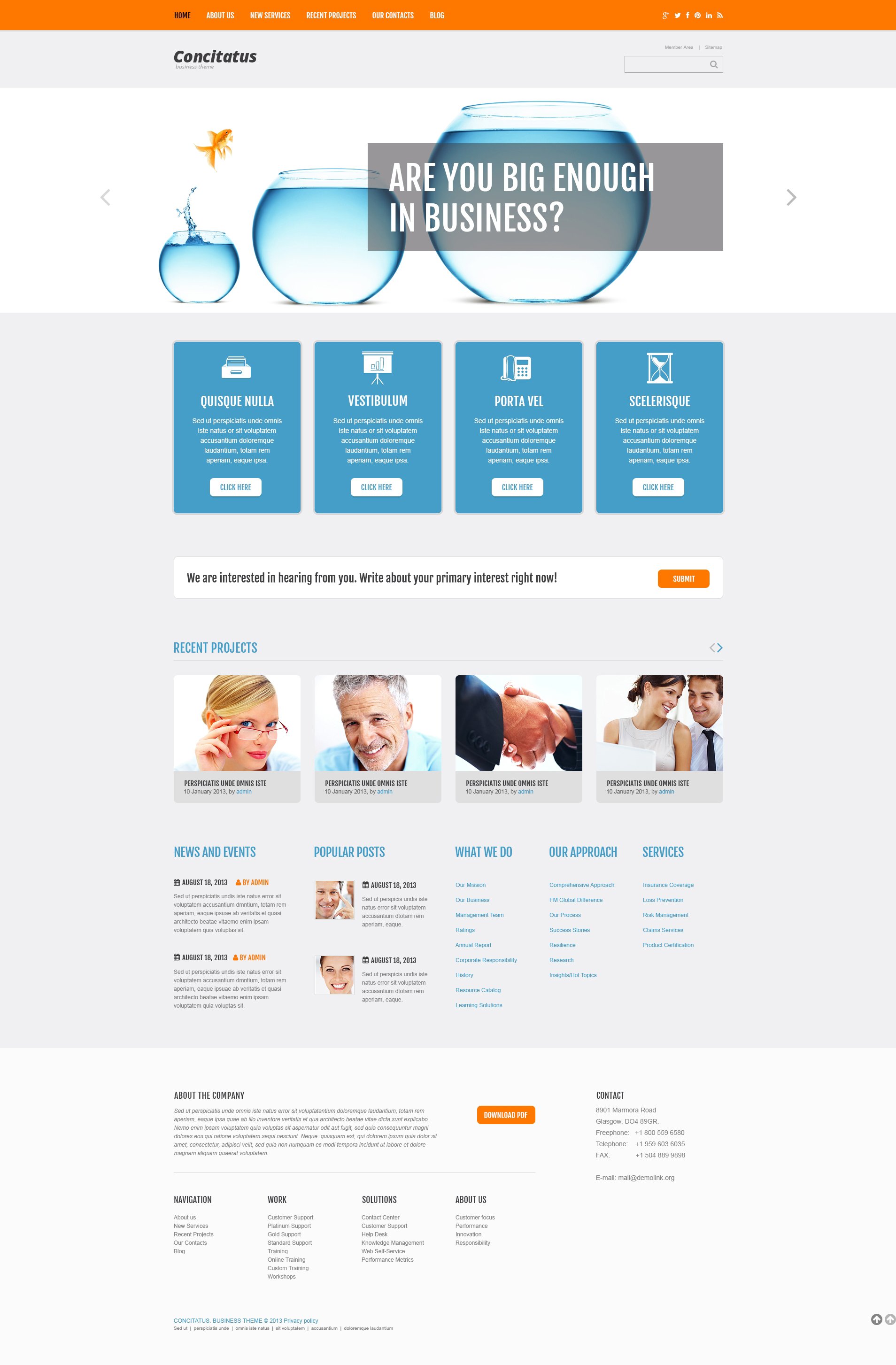This detailed caption describes a screenshot of the website "Concitatus":

*"The website for Concitatus, prominently displayed with bold black typography, features a striking visual theme. An orange stripe runs across the site, highlighting the primary sections. At the top of the page, three clear, round fish bowls of varying sizes are showcased, representing a dynamic visual progression. The bowl on the left is the smallest, followed by a medium-sized one in the center, and a very large one on the right. Each bowl is filled with water, creating a sense of balance and harmony. Remarkably, from the smallest bowl, a dramatic splash is depicted as a little goldfish leaps out, seemingly aiming for the medium bowl, symbolizing growth or transition.

Below this captivating imagery are four informative blocks labeled: Kisanella, Verastatium, Portovel, and Scarialisic, each likely providing specific details or sections of the site. A notable piece of text prompts user engagement: 'We are interested in hearing from you, write about your primary interests right now.' Complementing the layout, four images of people's interactions add a personal and relatable touch, encouraging visitor participation and connection."*